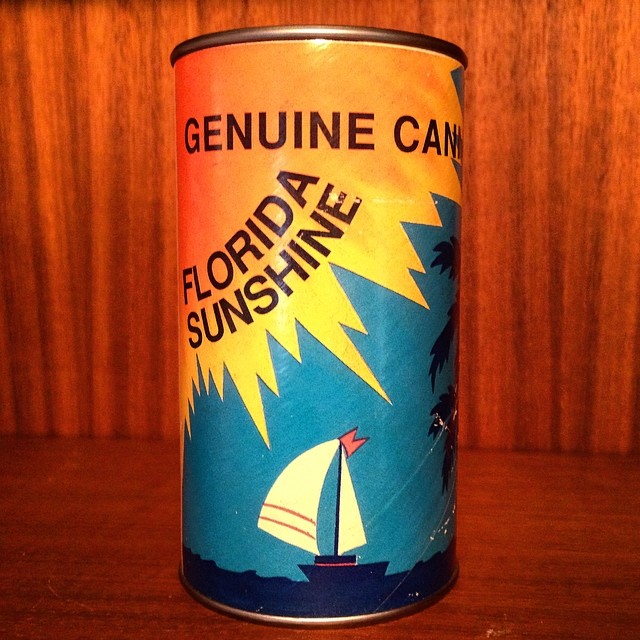This image depicts a can situated on a reddish-brown wooden surface, possibly a tabletop, with a matching wooden wall in the background. The can features exposed bare metal at the top and bottom ridges but is primarily covered by a detailed label. The upper left segment of the can's label showcases a bold clipart-style yellow sun with the words "Genuine Can" and "Florida Sunshine" in black text, curving to follow the sun's shape. The lower part of the label displays a light blue sky and a sailboat, which has white sails adorned with red and pink stripes and a pink crown, set against dark blue water. There are also dark blue palm trees visible towards the right part of the scene, complementing the design.